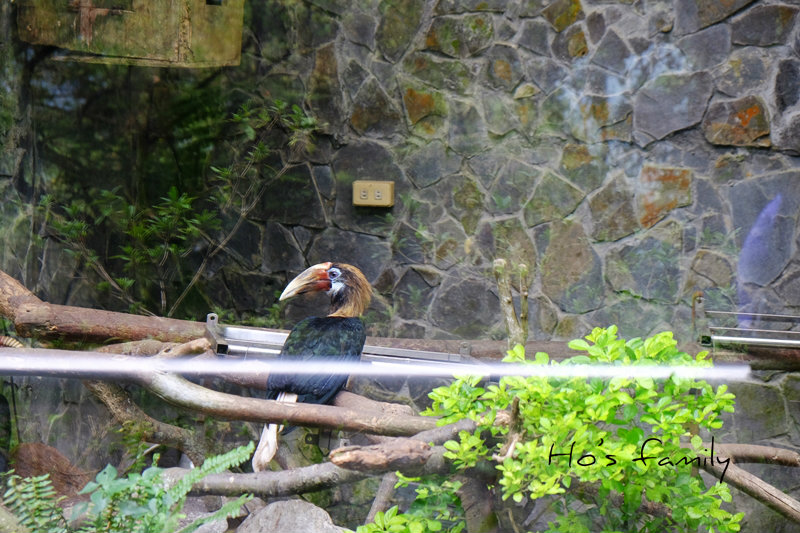This detailed, full-color photograph captures a significant-sized bird, likely taken outdoors, probably within a zoo enclosure. The bird, centrally positioned amidst some branches—some adorned with leaves and others bare—boasts a striking appearance with its black-feathered body, a brown and black neck, and a white patch under its cheek. Its beak is notable for its length and coloration, being cream-colored with accents of red and yellow. The background reveals a stone or brick wall characteristic of zoo environments, complete with visible electrical outlets centrally located on the wall. The bottom right corner of the image features handwritten text stating "Ho's family," suggesting ownership or the family associated with the photograph. The scene is set during daylight, as indicated by the vibrant colors such as brown, gray, tan, green, light green, red, black, and orange, which enhance the naturalistic feel of the outdoor setting.